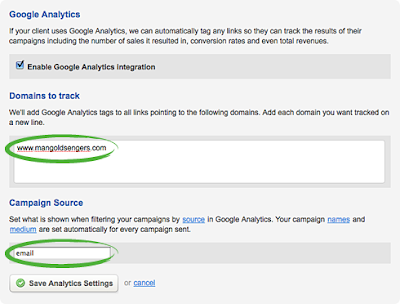The provided image features a comprehensive setup screen for Google Analytics integration filled with various instructional texts and interactive elements laid out on a light gray background. At the top, there's a drop-down menu labeled "Google Analytics," where "Google" is highlighted in blue.

Beneath, a note indicates, "Your client uses Google Analytics," followed by an explanation that the platform can automatically tag any links to track new campaigns, including metrics like the number of sales, conversion rates, and total revenues.

Below this, a dark horizontal box stands out with the text "Enable Google Analytics Integration," which is in gray and check-marked to indicate it has been enabled. Moving further down, a section titled "Domains to Track" in blue allows users to add the domains they wish to monitor. This section is followed by the instruction, "Add Google Analytics tags to all links pointing to the following domains." Listed beneath this instruction is a domain, "www.mangoldsingers.com," circled in green for emphasis.

Next, the "Campaign Sources" section, which is also highlighted in blue, provides configurations for filtering campaign sources within Google Analytics. Additional campaign properties like "Campaign Names" and "Mediums," both in blue text, are set automatically for every campaign.

Highlighted by another green circle is the text "email," within the "Campaign Sources" section, implying its importance.

At the bottom of the screen, there is a green check-marked button labeled "Save Analytics Settings," accompanied by a "Cancel" option as a blue hyperlink, providing a choice for users to either save their configurations or cancel the changes.

The overall design splits the interface into sections with subtle color differences between the light gray background and the slightly darker gray for the enabled features, guiding the user through the setup process.